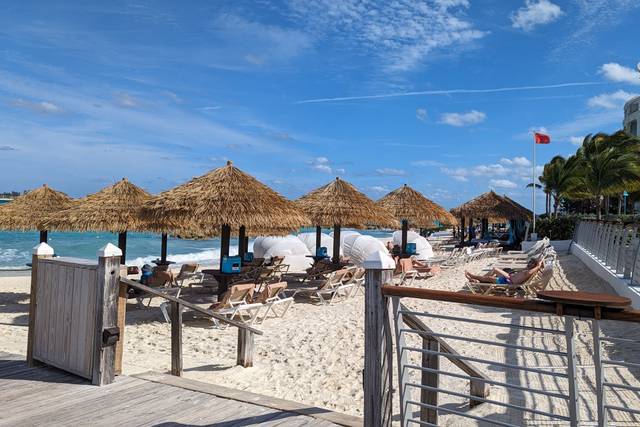This vibrant scene captures a sunny, tropical beach vacation spot viewed from the edge of a deck constructed with wooden boards, typical of a standard boardwalk. The deck features a white railing and a staircase that descends to a narrow strip of clean, light-tannish sand, dotted with long, folding beach chairs. Some of these chairs are occupied by beachgoers, some of whom are visible in hats, sunglasses, and bathing suits. Near the water's edge, there is a row of thatched straw umbrellas, each supported by wooden stakes, providing shade to the front-row beach chairs. The bright blue ocean is seen just beyond the umbrellas, with waves crashing onto the shore. A red flag on a white pole stands as a cautionary signal against swimming, likely due to toxins or rough weather. On the right side of the image, a few palm trees sway gently in the wind alongside a slightly visible gray building. In the background, a straw-thatched roof hut is seen at the far end of the beach. The sky above is a clear, bright blue with a few scattered, tiny white clouds, adding to the picturesque and idyllic nature of the scene.